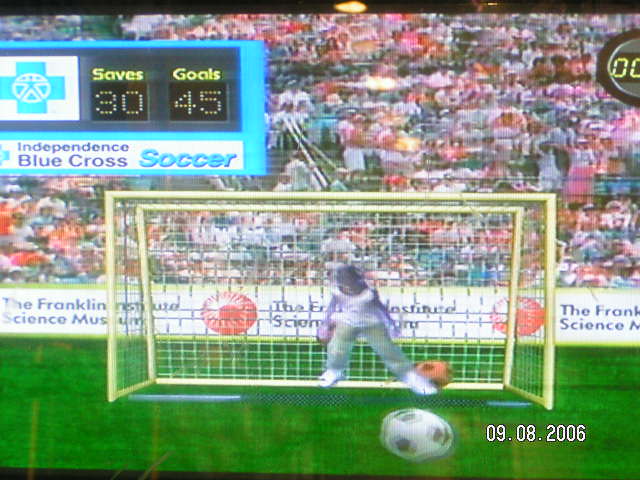The image is a blurry photograph showing a soccer scene, seemingly captured from a TV screen or monitor dated August 9th, 2006. The main focus is on a soccer field that occupies the lower third of the image, showcasing vividly green, thick, and healthy grass. At the center of the scene, a slightly washed-out child is positioned in front of a yellow soccer net. The child is flanked by two soccer balls—one red behind them and one white in front, as if a shot has just been made or missed. The top left corner of the screen displays text reading "Saves and Goals" and "Independence Blue Cross Soccer," indicating that it is a soccer game broadcast. The background depicts a large crowd, but the entire image is heavily blurred, suggesting motion or poor image quality.